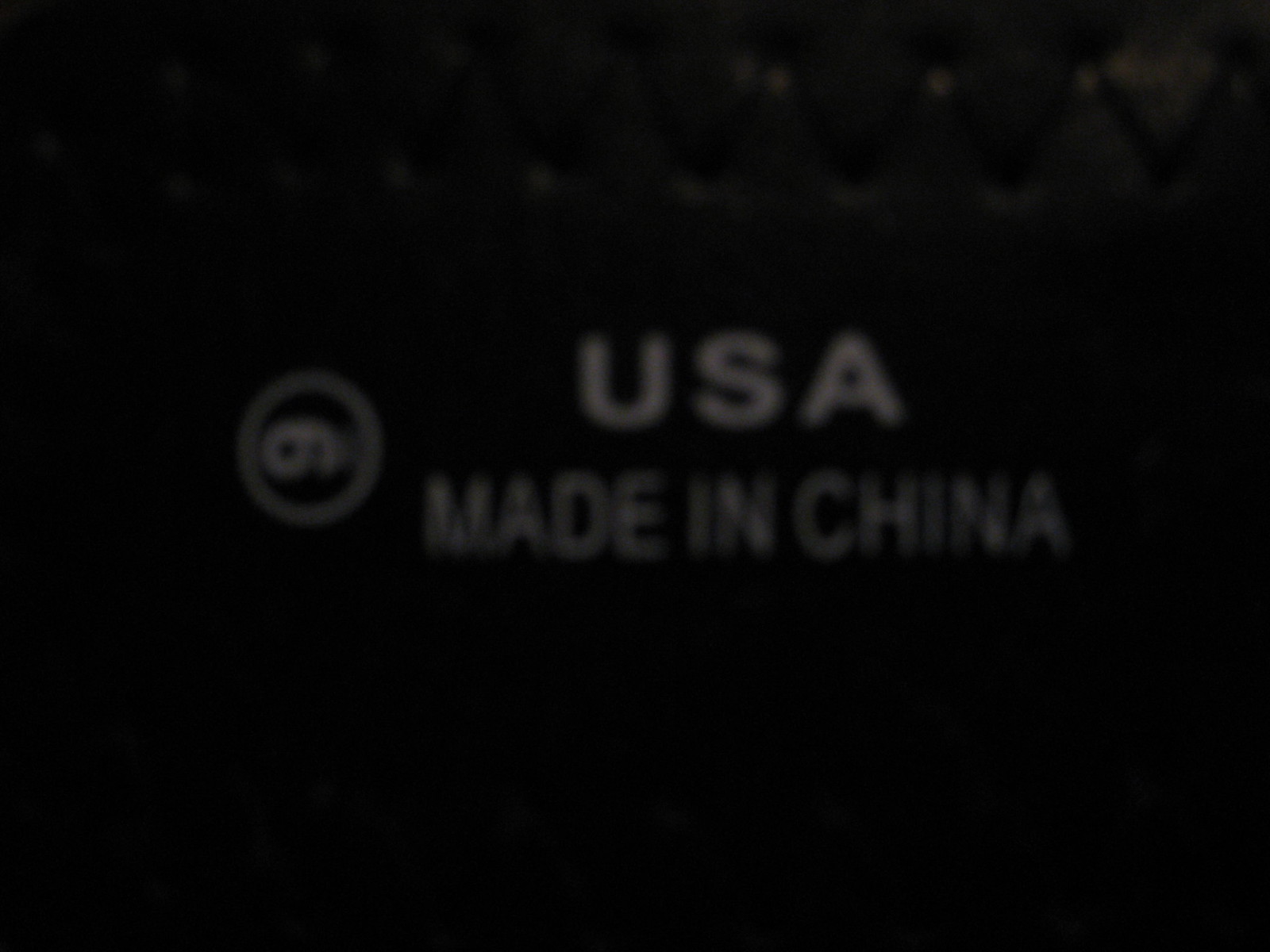This black and white image captures a close-up view of a clothing label in stark contrast against an almost completely black background. At the upper part of the image, three distinct dots are positioned near the right corner, extending about a third of the way in. Below these dots, there is another line of dots that stretches from the right corner to slightly past the halfway point. Adjacent to the far-right dot, a discernible smudge is visible. 

Beneath these dots, white print is present, featuring a prominent circle enclosing a number that might be a six or a nine, depending on the viewing angle. Following this, the text “USA” is clearly printed in white. Directly below that, the phrase “Made in China” is displayed, presenting a stark contrast and adding an element of irony to the label. The image, likely taken in poor lighting, focuses tightly on the details of the label, suggesting it is part of a clothing item.